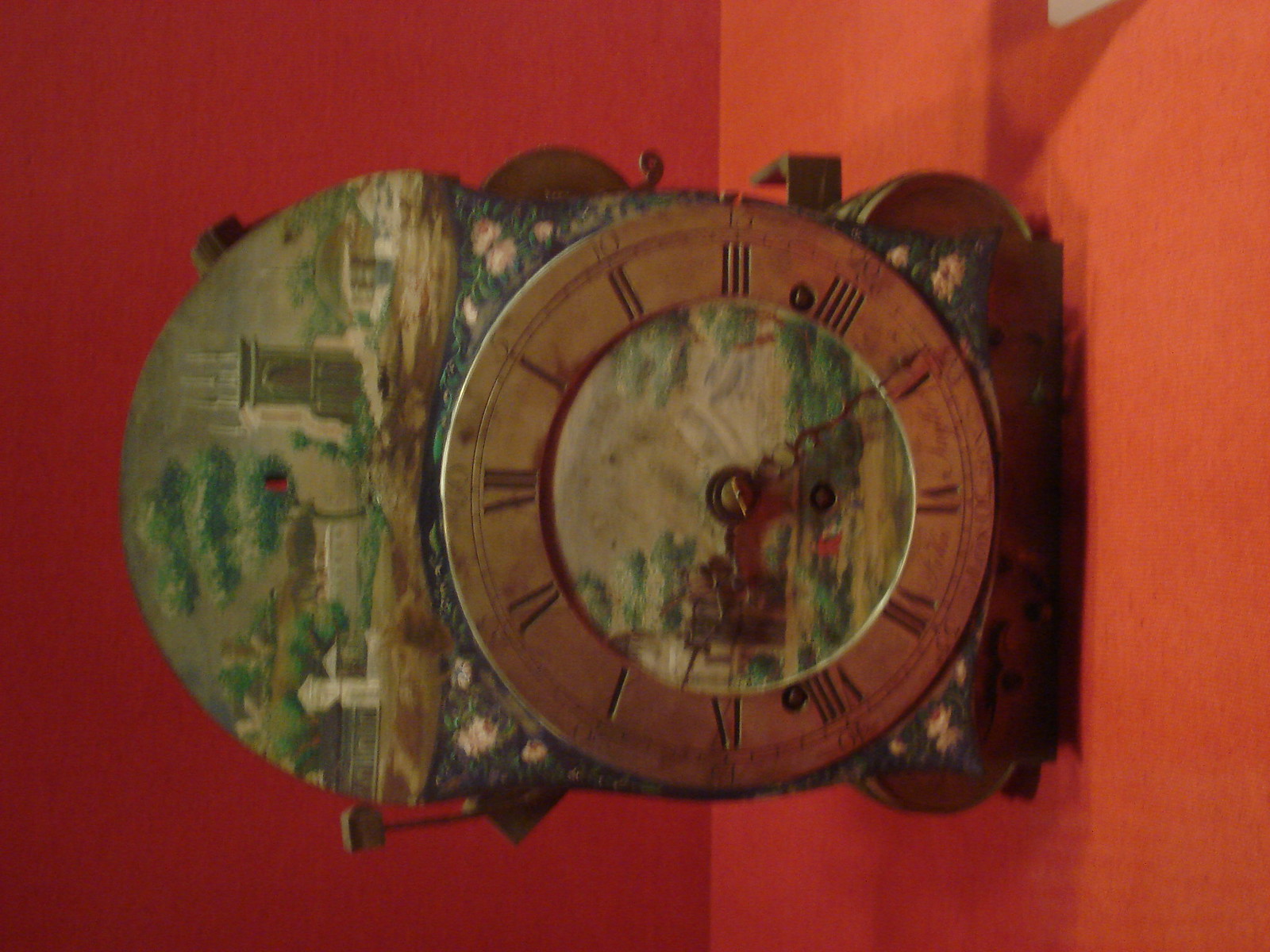This is a colour photograph of a vintage painted clock, which is inaccurately oriented in a landscape format. To view the clock correctly, the image should be rotated 90 degrees clockwise. The clock itself is designed to stand upright, rendering it in a portrait orientation.

The clock face is analogue and framed by a bronze band featuring engraved Roman numerals filled with black paint. Contrary to modern clocks, it lacks a second hand and only includes an hour hand and a minute hand. Dominating the interior of the clock face is a hand-painted water scene replete with trees, bushes, and a small bridge, suggesting a serene natural setting. The painting, seemingly crafted rather than mass-produced, lends an artistic charm to the piece.

Further inspection reveals that around the circumference of the clock's face, a grey, weathered ring showcases the Roman numerals. Above the clock face, part of the clock's mechanics is visible, including a small hammer indicating an hourly chime feature. The entire scene rests on a red table against a matching red background, but the blurred quality of the image makes it challenging to ascertain finer details, including the specific scenes painted on the clock's body, which appear to include depictions of a doorway and trees.